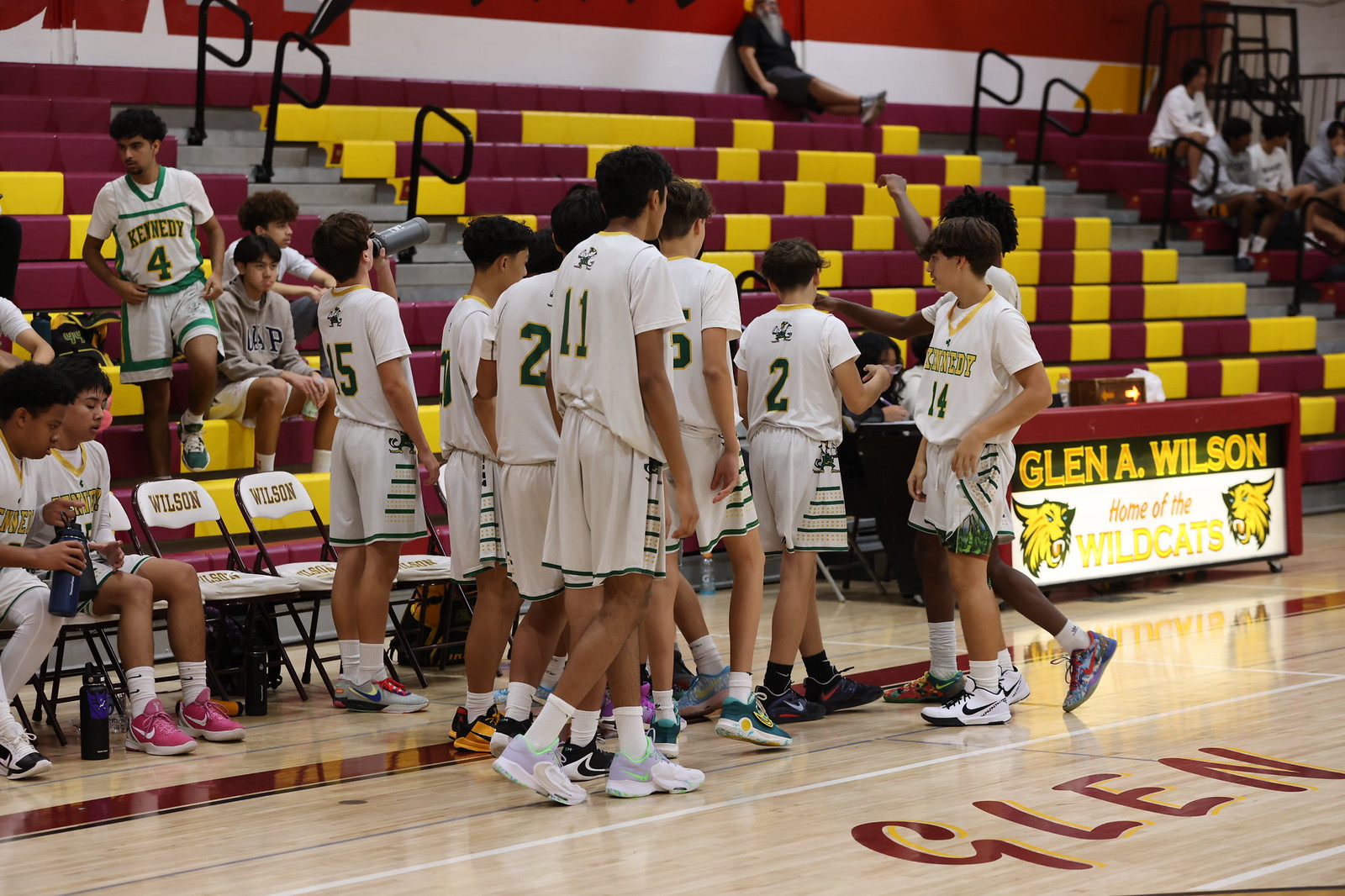This vibrant photograph captures a high school basketball team during a game at Glenn A. Wilson, home of the Wildcats. The gymnasium features rows of yellow and maroon-striped bleachers with minimal spectators. At the forefront, several young teen boys, possibly aged 12 to 14, are gathered around their coach, preparing for a high-five. They are dressed in white jerseys and shorts, with numbers in green outlined in yellow, including 2, 11, 14, 15, and 4. Some players are seated in folding chairs marked with "Wilson," while a banner at the scorer's table proclaims "Glenn A. Wilson, Home of the Wildcats" flanked by images of Wildcats. The image is brightly lit, highlighting the energetic and supportive atmosphere as the team engages in their sport.